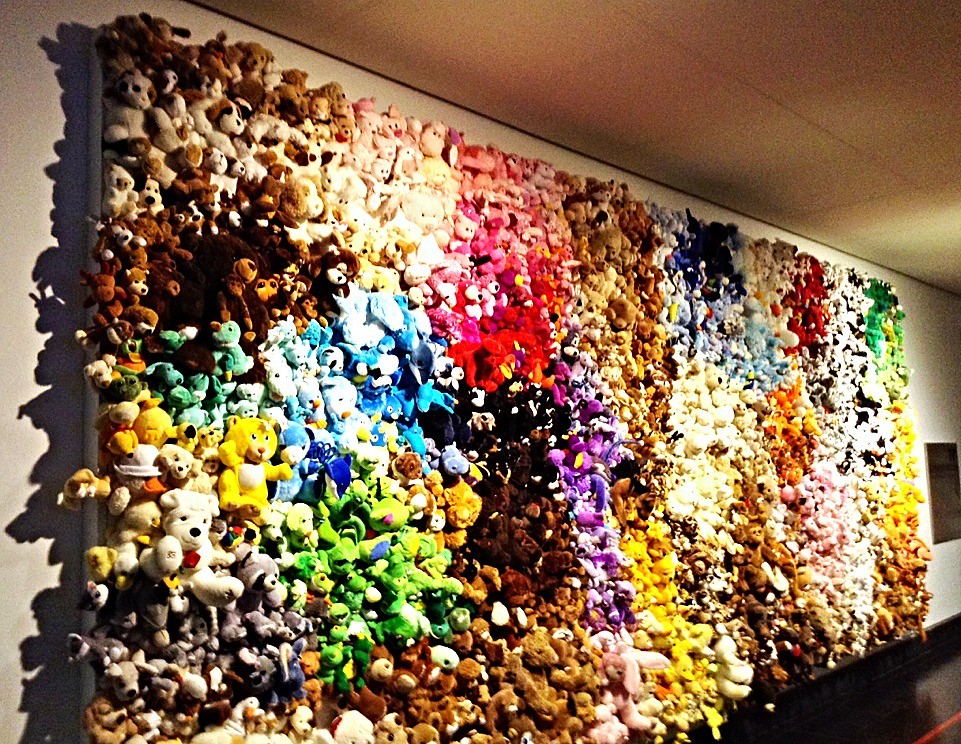The image features an expansive art installation that spans an entire wall, resembling a massive canvas of small stuffed animals densely packed together. Each section of the wall is color-coordinated, with different parts occupied by groups of varying hues and types of stuffed creatures. At the top right, there are clusters of brown and white dogs, followed by rows of brown bears. Progressing through the canvas, there are green dogs, yellow teddy bears, and other colorful assortments, including pink, red, purple, and blue stuffed animals. Among these are distinct shapes resembling frogs or alligators, as well as monkeys, all intricately interwoven yet arranged in specific color blocks. The overall piece is as tall as an average wall and nearly as wide as a car, making it an impressive exhibit that would be a captivating sight in any art museum.